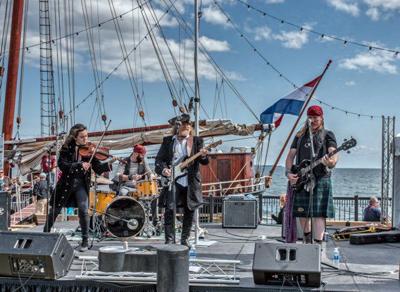In the image, a lively band dressed as pirates performs on the deck of a large old ship. Featured prominently are three musicians: a woman on the left playing a violin, a man in the middle holding a guitar, and another man on the far right also with a guitar. The violinist and the guitarists have microphones in front of them, singing passionately into the blue, almost cloudless sky. Behind them, another band member is seen playing the drums.

The scene suggests they might be docked at a pier, as indicated by a significant pillar that could be part of the dock. The ship's massive sail and towering mast emphasize its grand scale. Large speakers are positioned in front of the band to project their music. It's a bright midday, perfect for an outdoor performance, with the clear ocean water visible in the background. A person is seen on the other side of the ship, possibly sitting and watching the water, adding to the serene yet festive atmosphere. Water bottles are scattered at the musicians' feet, ensuring they stay hydrated during their energetic performance. The band’s costumes, including one member dressed in an Irish skirt, contribute to the thematic pirate concert ambiance.